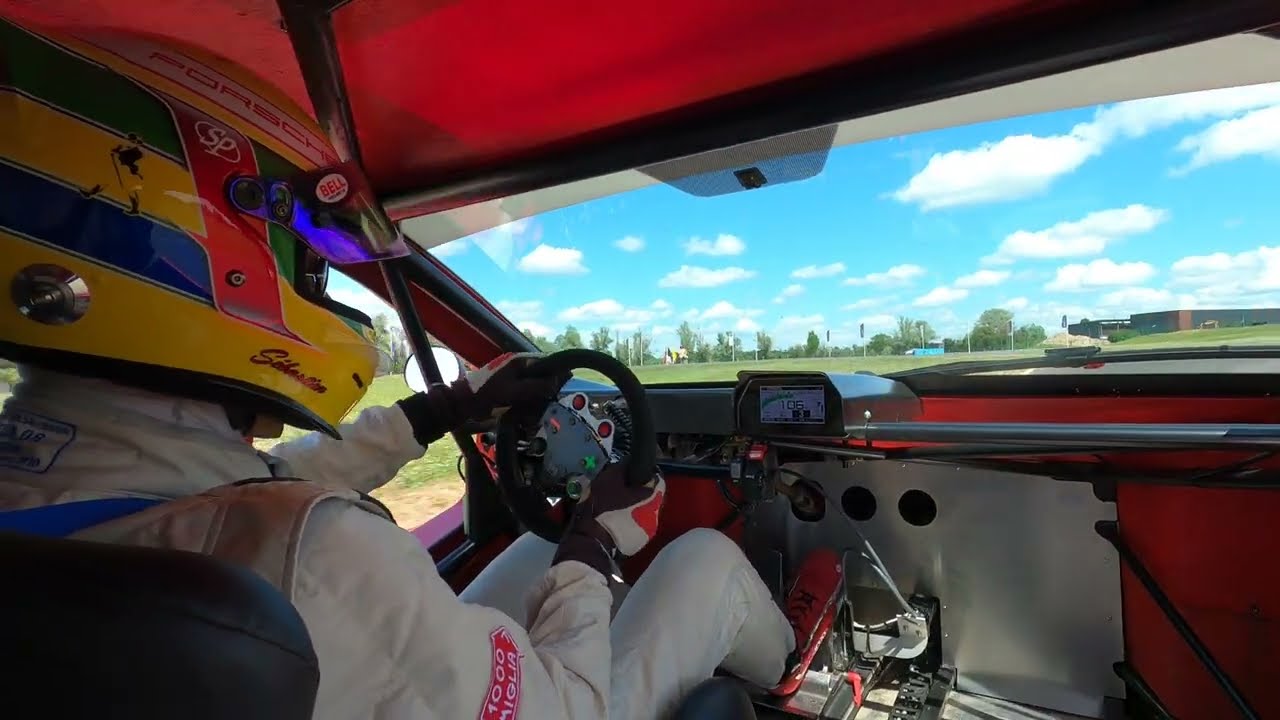The detailed image captures the interior of a race car, providing a view from slightly over the shoulder of the driver. The car's body is predominantly red and possesses a slight translucence, allowing light to filter through the ceiling. The interior is minimalist, featuring only a speedometer and a steering wheel in the driver's compartment. The driver is donned in red tennis shoes, a white race suit, and has a red and white patch on their right arm. They are wearing a yellow helmet adorned with blue and green stripes, along with a prominent white stripe that reads "Porsche" in red font. The helmet's visor is flipped up, revealing the driver’s face. Both of the driver’s gloved hands are firmly grasping the steering wheel as they navigate a right turn. The environment outside hints at a sunny day, emphasized by the light streaming into the vehicle. On the speedometer, the car's speed is gauged at 106 miles per hour.